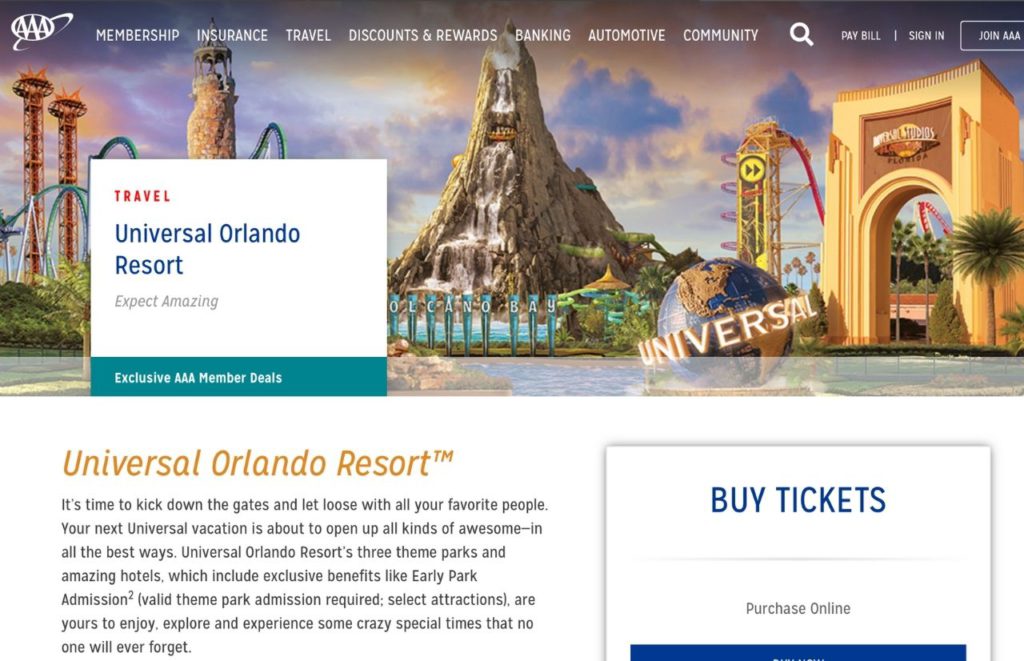The image displays a section of the AAA website. In the upper left corner, the distinctive AAA logo is visible, featuring three "A" letters within an oval, which itself is tilted at an angle. Adjacent to the logo, the website's menu lists the categories: "Membership," "Insurance," "Travel," "Discounts & Rewards," "Banking," "Automotive," and "Community." To the right of the categories is a thick, bold magnifying glass icon indicating a search function, accompanied by options to "Pay Bill Online," "Sign In," and "Join AAA," all within a semi-transparent rectangle that blends seamlessly with the website's media background.

The media image prominently displayed behind this menu features a picturesque mountain scene reminiscent of Universal Studios. The iconic Universal Studios globe, with "Universal Studios" written in bold, traditional letters, is superimposed over the mountain image. Visible are a few theme park rides, including what appears to be a roller coaster, partially obscured by text.

The main banner reads "Travel Universal Orlando Resort," with a subheading "Expect Amazing." Below this, an aqua blue banner announces "Exclusive AAA Member Deals," followed by "Universal Orlando Resort." A paragraph of text related to these deals is partially visible. On the right side of the image, there is a section labeled "Buy Tickets" and "Purchase Online," although a blue rectangular box is cut off, partially hiding details.